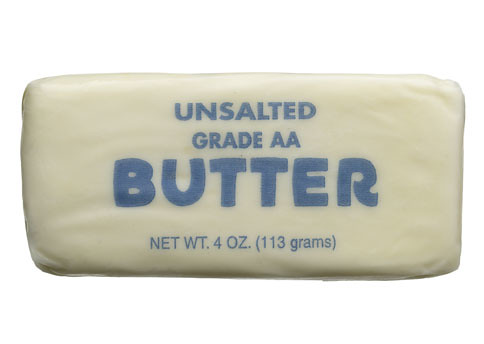Here is the cleaned-up and detailed descriptive caption:

"A photograph of a rectangular brick of unsalted Grade AA butter is prominently displayed in the center of this image. The butter, weighing 4 ounces or 113 grams, is neatly wrapped in wax paper. The packaging features text in a distinctive cornflower blue color. The backdrop of the image has been digitally whited out, causing the butter to appear as if it is floating in an empty space, drawing full attention to the simplicity and clarity of the product's presentation. The overall visual effect emphasizes the purity and quality of the unsalted butter."